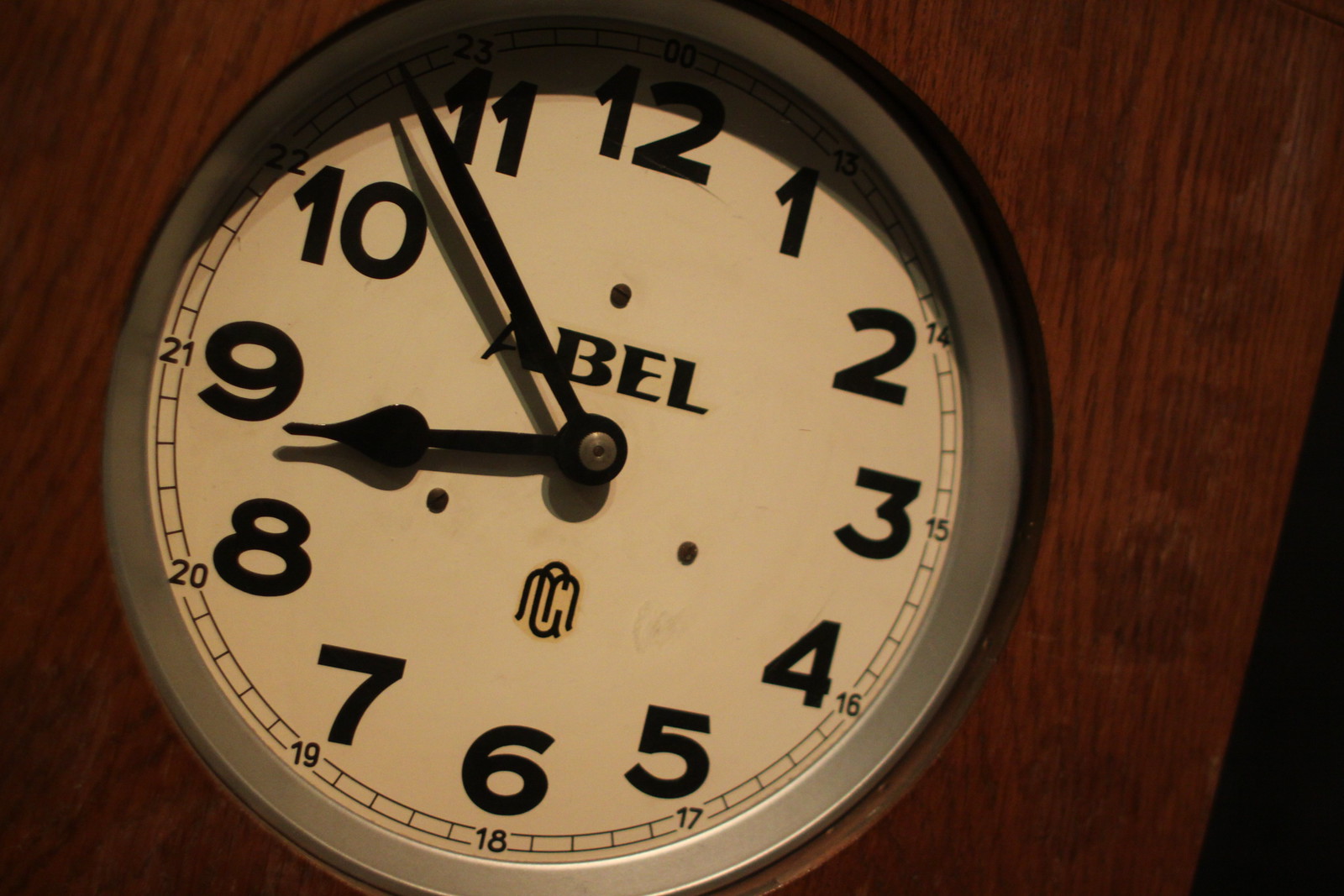The image features a traditional-looking, circular clock prominently displayed against a wooden background, which could be either a wood-paneled wall or a wooden table. The clock has a white face with bold, black sans-serif numbers ranging from 1 to 12, and additional 24-hour markings at the periphery. Its rim consists of a black case with a gray inner circle. The clock indicates the time as 8:54. There are small marks for each minute, and the brand name "Abel" is clearly visible near the top center of the clock face. The setting appears somewhat dark, accentuating the fine grain of the wood and casting a subtle shadow on the upper part of the clock. A small sliver of black is noticeable to the right side of the image, but the main focus remains on the clock itself, with its clear, crisp design.